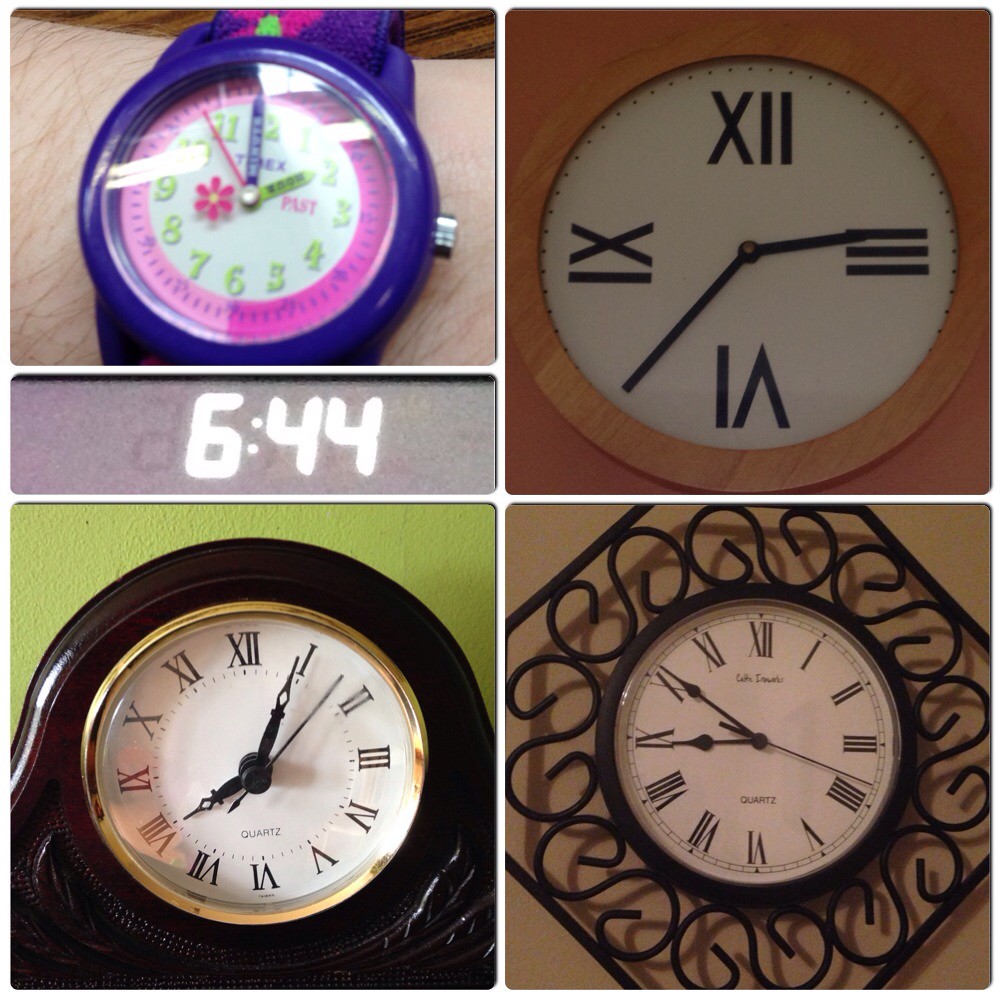This image is a collage consisting of five distinct photos, intricately arranged to display a variety of timepieces. In the top left corner, there are two photos creatively merged together: one features a digital clock showing the time 6:44, and the other showcases a bright pink and green children's watch adorned with floral designs. Moving to the top right, another clock is depicted, but only the positions of four numbers are visible, offering a minimalist view. The bottom left photo reveals an old-fashioned alarm clock, evoking a sense of nostalgia. Lastly, the bottom right image displays a classic wall clock, neatly hung and sporting Roman numerals. It's noteworthy that all the clocks on the right side and the bottom left exhibit Roman numerals, while the two in the upper left corner present either digital or standard numerical formats.